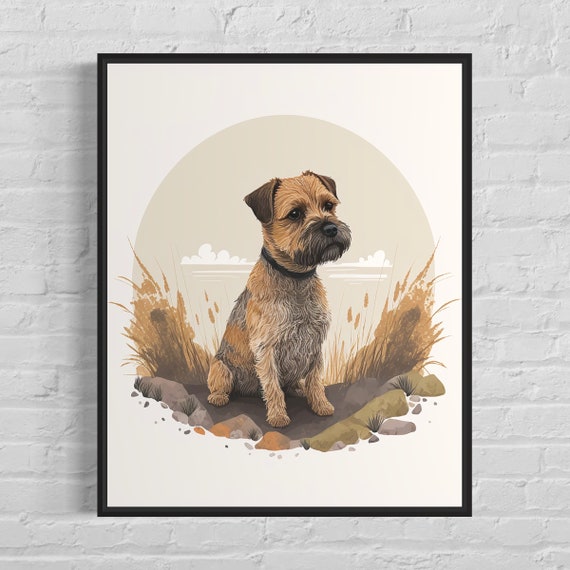The image is an artist's print or digital painting featuring an adorable, small brown dog that resembles a mix of a terrier, possibly a Brussels Griffon and a schnauzer, with some characteristics of a Westie. The dog has dark brown ears, a darker brown muzzle, a black nose, and dark brown eyes. It wears a black collar and sits in a charming pose with its hind legs and rear on the ground, front legs propping it up, gazing off into the distance with a pensive expression. The background includes a patch of dirt and rocks, sprouting some yellow grass or wheat, giving it a natural, serene feel. The framed artwork, encased in glass, is displayed on a grayish brick wall, adding to the rustic and peaceful ambiance of the scene.